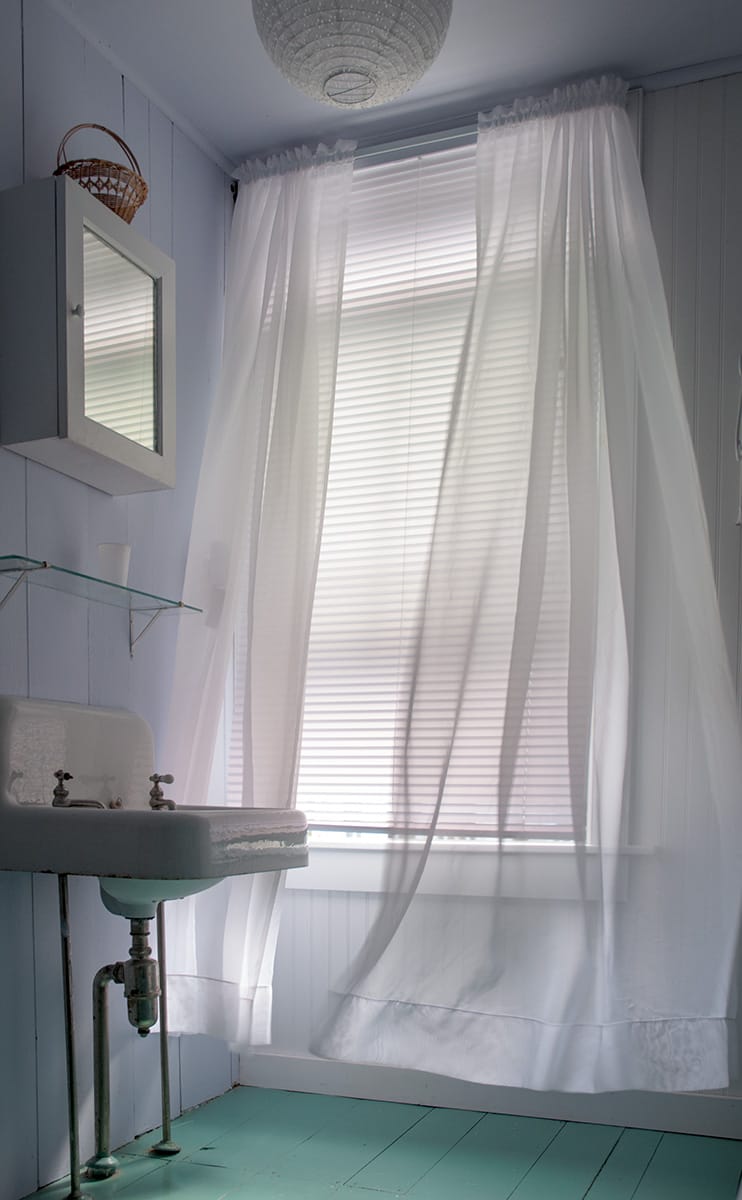The image depicts an old-fashioned bathroom with a teal green linoleum floor. The focal point is an open sink with exposed intake pipes and two separate faucets, evoking a 1950s design. Above the sink is a small glass shelf with a single plastic cup, and further up, a mirrored medicine cabinet, topped with a brown basket. The medicine cabinet is mounted on a light purple wall. The window, partially obscured by light gray blinds and see-through white curtains, suggests an opening behind the blinds as the curtains are gently billowing. There is a potential smoke detector or another small object on the ceiling in front of the window. The right-hand and lower portions of the image include gray walls, intensifying the room’s vintage look.